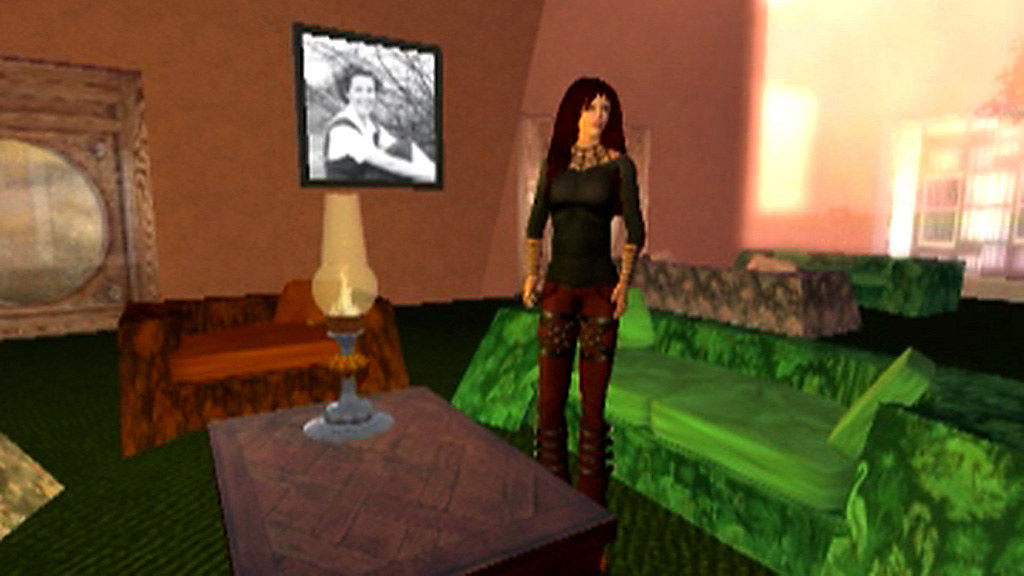In a simulated lifestyle game, a tall, slender woman with long black hair stands in a stylish living room. She wears a long-sleeved black shirt featuring high cuffs in brown, paired with tight-fitting brown pants which have a distinctive design on the thighs, and she completes her ensemble with boots. She is positioned in front of a kelly green couch, adding a touch of vibrancy to the room. A brown low coffee table is situated in front of her, holding a lantern-style lamp that emits a warm glow with visible flickering flames inside the vase. The walls are painted a peachy pink hue, balancing the room's color palette. Adorning the wall is a black and white framed photograph capturing a woman seated on the ground with her knees pulled up to her chest and her arms wrapped around them. The woman in the photograph, who appears to be wearing a school uniform, smiles warmly at the camera, while a backdrop of bare trees enhances the nostalgic feel of the setting.